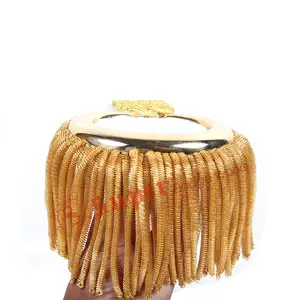The image depicts a gold-fringed epaulette, often used in uniforms for decoration, resting on a white background without borders. The epaulette features intricately detailed, segmented tassels of a tan to light brown color base, resembling tubes or strands that hang down vertically and appear to be hollow in the center. These tassels encircle the base entirely, giving the impression of dense, worm-like fringes. Adding to the complexity is a visible round base with a metal underside and a white strap across its center, hinting at the structured design of this uniform accessory. In the foreground, a Caucasian hand holds the epaulette, providing a sense of scale and placement within the frame. Red lettering is digitally added to the image, but it’s indecipherable.